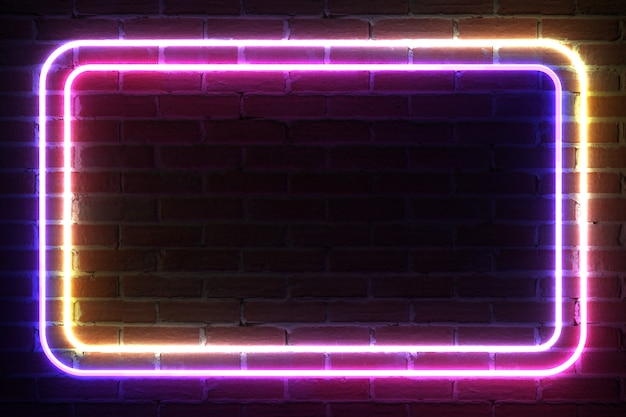The full-color photograph, likely taken indoors with artificial lighting, is horizontally rectangular with no border. It showcases a darkened red brick wall, with approximately 15 rows of bricks visible. The center of the wall features a striking neon frame composed of two horizontally rectangular neon lights. The larger light transitions from a yellow hue on the top and right to a purplish color on the bottom and left, while the smaller light inversely shifts from yellow on the lower right to purple on the left. The neon lights emit a bright, strong color, creating an illuminated border around the center of the wall, which remains dim and unadorned, evoking an invitation for adding a logo or other objects.